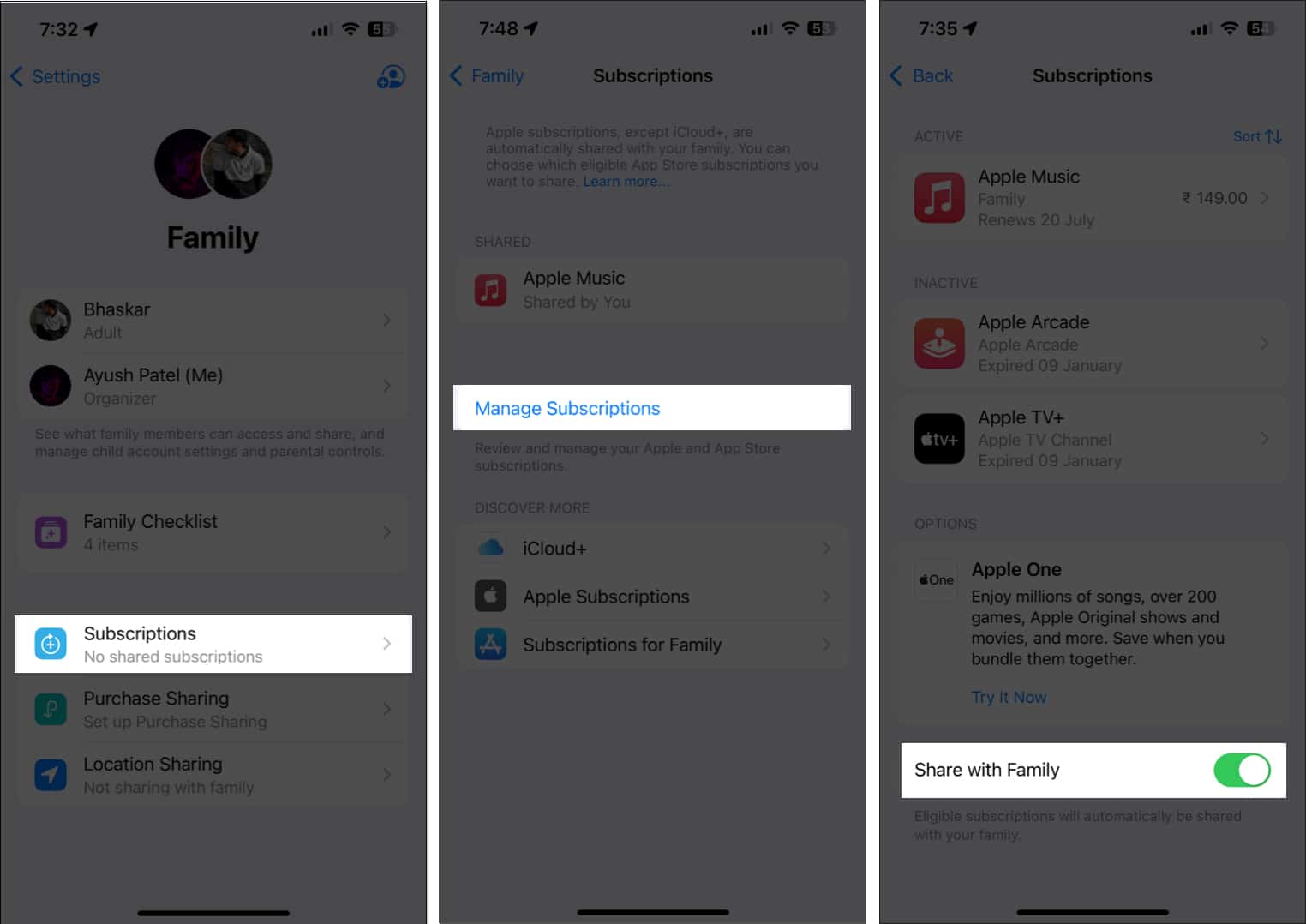This image is divided into three sections, each displaying a different phone screen. The screens are overlaid with a semi-transparent gray color, making the text slightly difficult to read.

The leftmost phone screen shows a time of 7:32 in the upper corner. It features a back arrow labeled 'Settings'. Below, there are two circular profile icons with the heading 'Family'. The first profile, labeled 'Bhaskar', is identified as 'Adult'. The second profile features 'Ayush Patel', marked as 'Me, Organizer'. Beneath these profiles, there's text that informs about the family members' access and sharing settings within 'Parental Controls'. Additionally, there's a 'Family Checklist' where the item 'Subscriptions' is highlighted, showing 'No shared subscriptions'.

The middle phone screen displays a time of 7:48. The header of this screen reads 'Subscriptions'. Underneath, it mentions 'Shared Apple Music, shared by you'. Importantly, a 'Manage Subscriptions' option is highlighted within a box.

The rightmost phone screen shows a time of 7:35. It also has a header labeled 'Subscriptions'. The screen is divided into sections for 'Active' and 'Inactive' subscriptions. Under 'Active', it lists 'Apple Music, Family, Green News' with a date of '20 July' and a symbol followed by '149.00'. The 'Inactive' section lists 'Apple Arcade' and 'Apple TV Channel', both expired on '09 January'. At the bottom, there's an 'Options' section where 'Apple One' is mentioned and the option 'Share with Family' is highlighted and enabled.